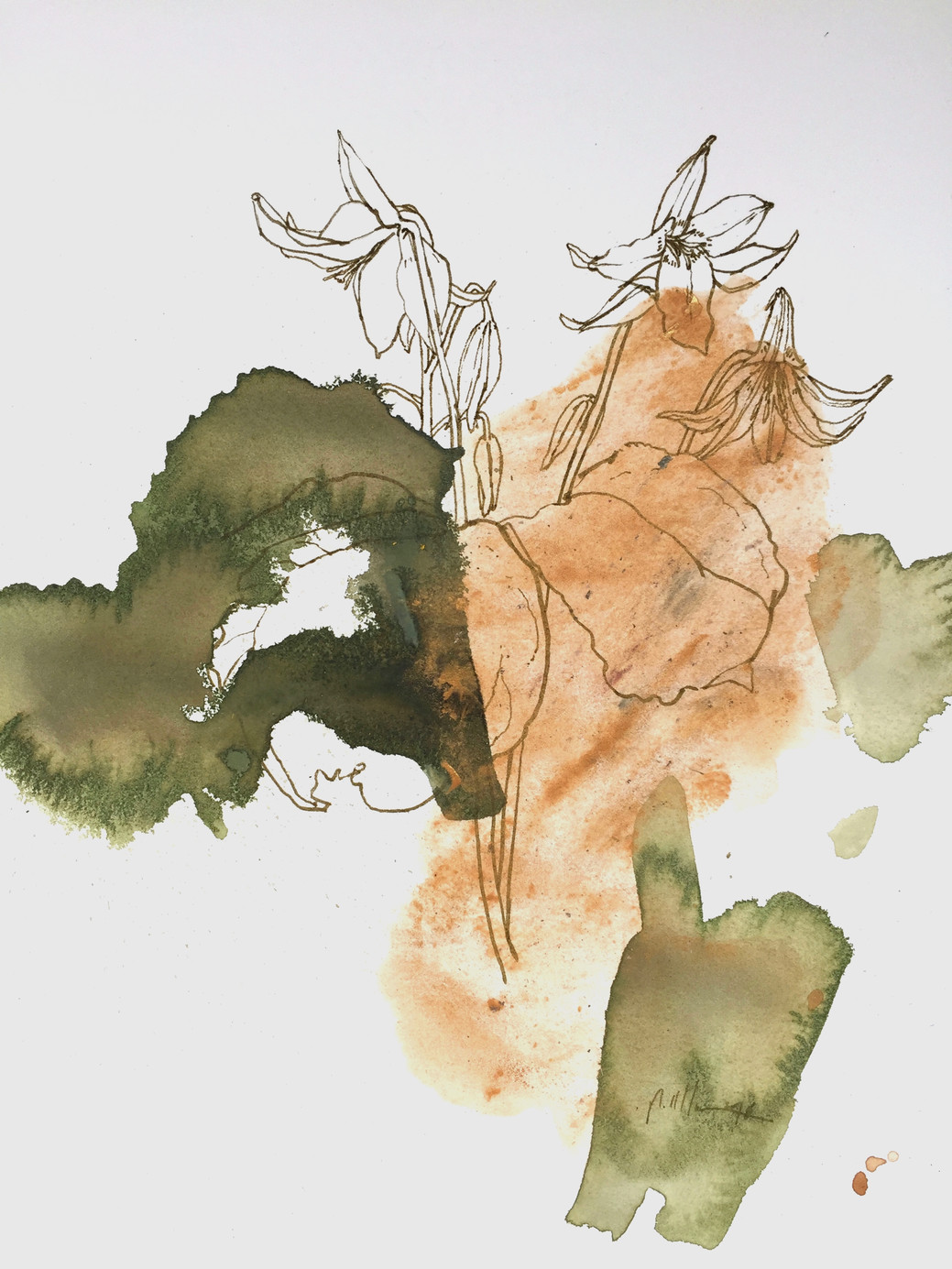This is a photograph or scan of a hand-drawn set of flowers on a white background, featuring a striking blend of chaotic yet intentional paint smears. The stems rise upwards into leaves and flower petals, prominently adorned at the top with several blue flowers. These flowers have additional layers of vibrant colors painted over them. The background appears light gray, adding a subtle contrast to the foreground elements.

In the center right, a swipe of orange paint stands out in a smear pattern across the piece. Beneath it and towards the bottom, green splotches dominate—most notably, there's a large green splotch with the artist's signature on top, indicating the creator's mark. The left side of the image features a darker green stain that extends over the flowers and leaves, giving the piece a dynamic asymmetry.

Tiny red splotches are visible in the bottom right corner, adding another layer of color detail. Light tan paint is present predominantly in the center of the image amid the flowers, with a larger flower at the front and center offsetting the background blooms that mostly point upright, except for one wilted and tilting flower on the far right. This intentional and wild overlay of paints—ranging from olive green to light brown—over the floral sketches suggests a deliberate artistic style aimed at blending chaos with the delicate line work of the flowers.